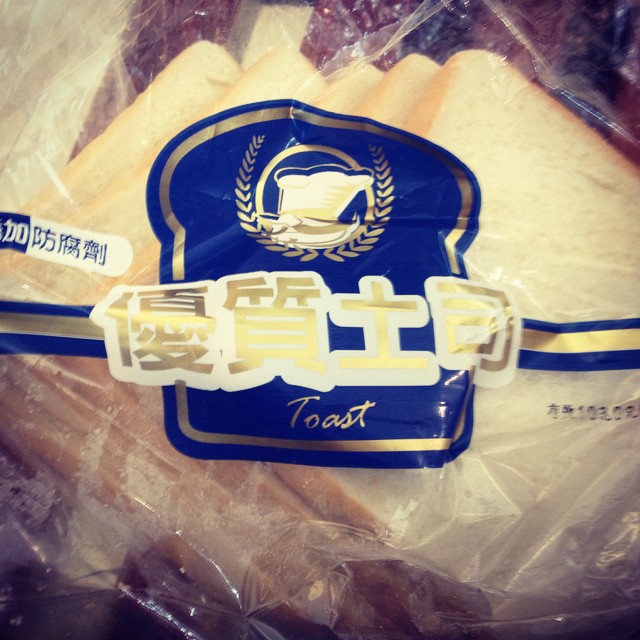This close-up photograph features a transparent, cheap-looking plastic bag containing at least five to six slices of white bread. The bread slices, which have a light brown crust typical of white bread, are not neatly stacked and some appear to be separated. The bag has a distinctive blue-colored label, trimmed in gold, which is shaped like a piece of toast. This label prominently displays a stylized gold emblem of wheat in a circle beneath an image of a slice of bread. Below this is the word "TOAST" written in gold cursive script. Additionally, the label includes gold calligraphy script, likely in either Japanese or Chinese. To the left and right of the label, more character writing in blue and white can be seen, including a blue rectangle with white calligraphy in the upper left corner, and a date stamp indicating when the bread should be consumed on the right-hand side.